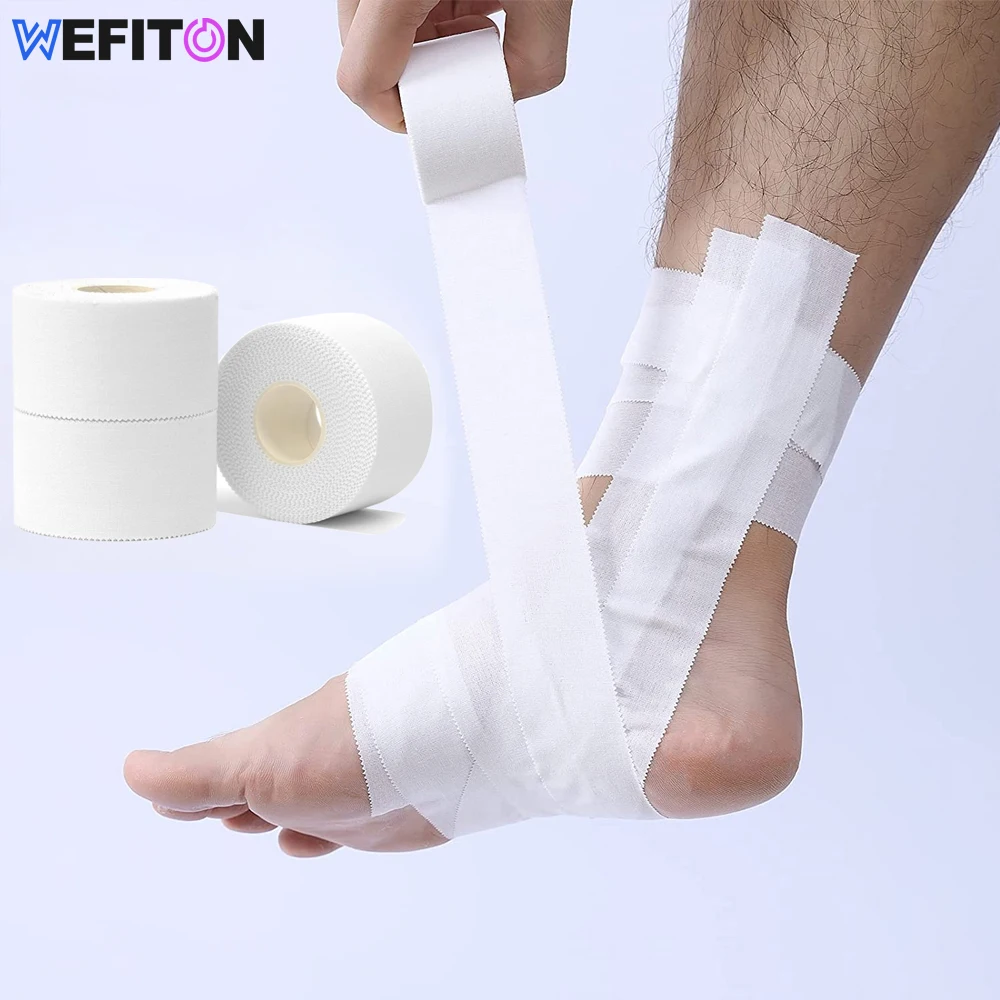The image features a light blue background and prominently displays a man's hairy leg, shown from mid-calf down, as he wraps white medical tape around his foot and ankle, excluding the heel and toes. In the upper left corner, the logo "Wefiton" is displayed with a blue "W", a purple "O", and the rest of the letters in black. To the left of the foot, there are three additional rolls of the white medical tape.